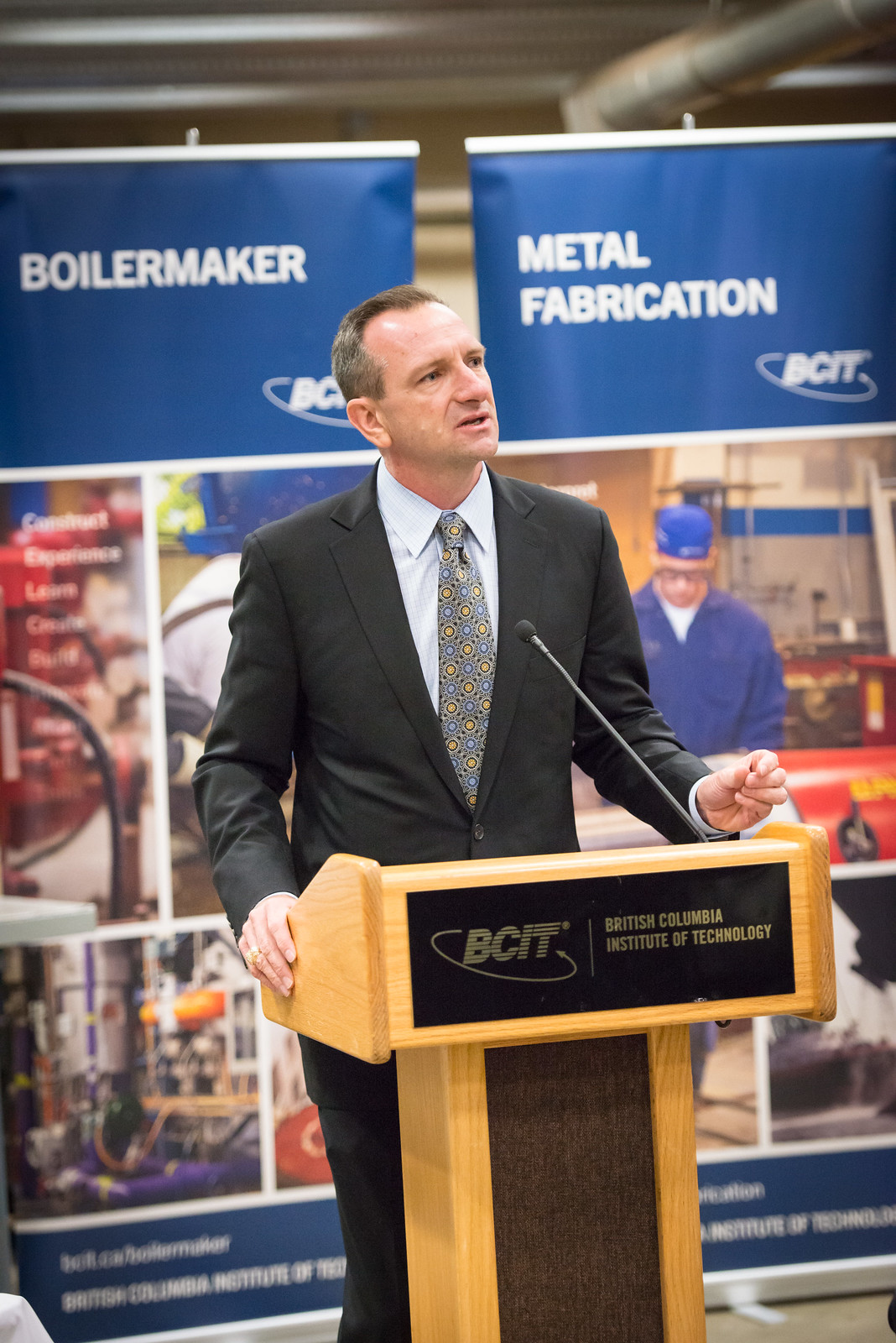The image depicts a white male presenter standing at a wooden podium, made of light wood, with a microphone extending from the top. The podium features a black plaque with yellow text that reads "BCIT" and also spells out "British Columbia Institute of Technology." The man is attired in a black suit paired with a light blue dress shirt and a patterned blue and yellow tie, and he has short brown hair and a receding hairline.

Behind him, there are two blue banners with white text. The left banner reads "Boilermaker," and the right banner reads "Metal Fabrication." Both banners include images depicting industrial work and have "BCIT" in the bottom right corner, reinforcing the focus on trade skills education. The venue where he is speaking appears to be indoors, likely part of a conference or a convention aimed at showcasing the educational opportunities and programs at the British Columbia Institute of Technology related to boilermaking and metal fabrication.